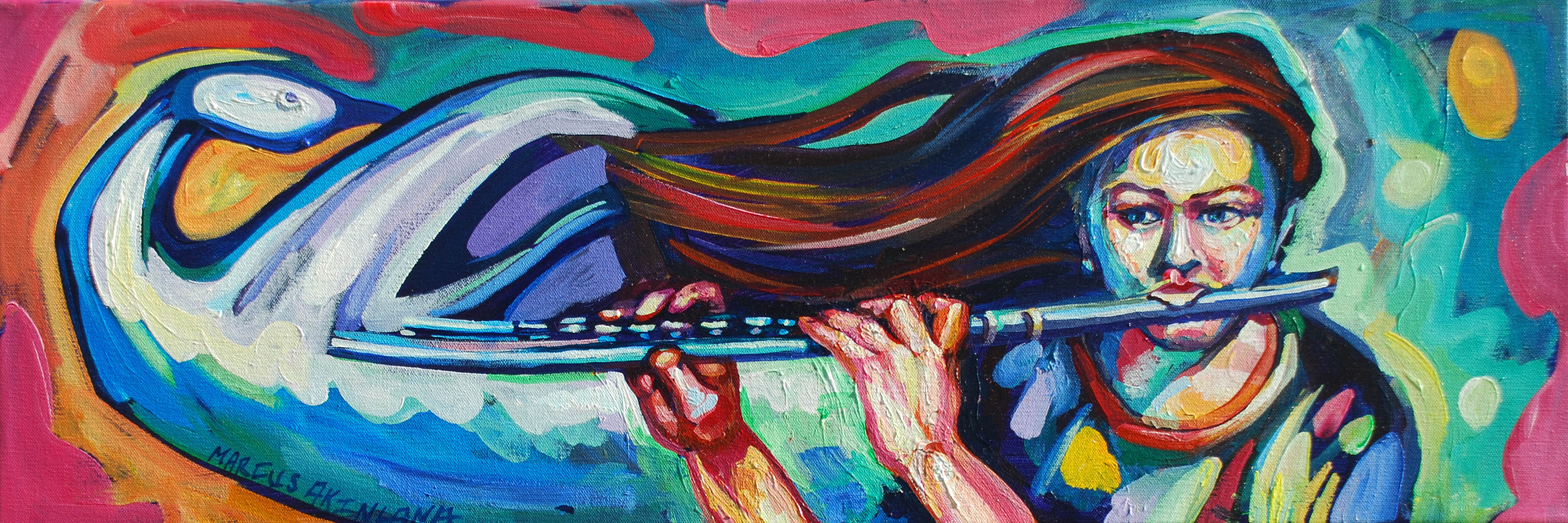The painting features a woman with flowing, rainbow-colored hair, which includes shades of brown, red, blue, yellow, and purple, blowing in the wind as she plays a long, metallic flute. Her hands are positioned on the flute, and her mouth is wrapped around it, suggesting she is deeply immersed in the music. The woman is dressed in a shirt adorned with a vibrant array of colors, including navy with pink, green, yellow, blue, and purple spots. The background is equally colorful and dynamic, with swirls of blues, whites, reds, oranges, pinks, and greens, and it even features a swan-like shape on the left side. At the top of the painting, the name "Marcus" is prominently displayed.